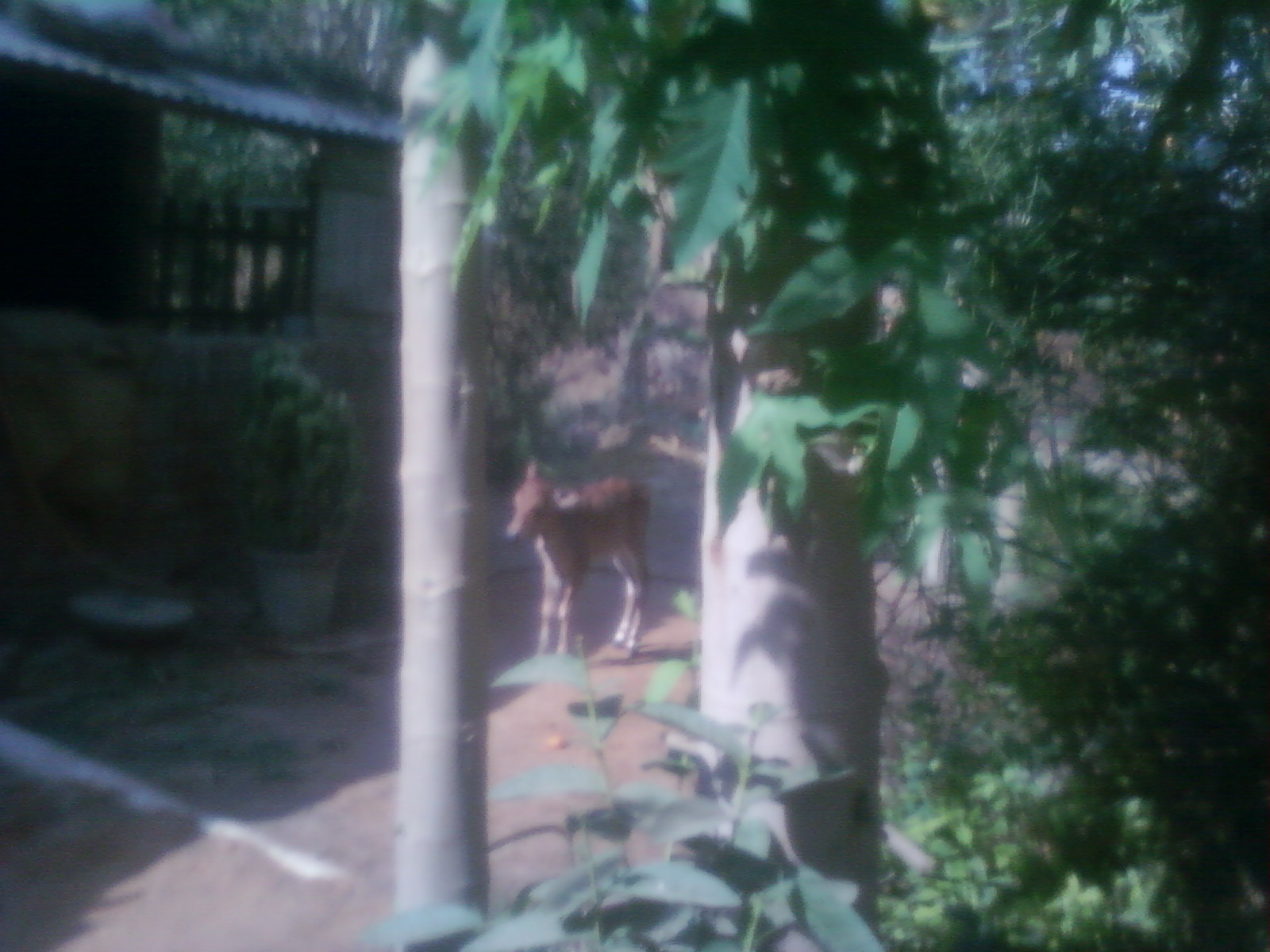The daytime photograph captures a slightly blurry outdoor scene. On the right side, an array of tree trunks, abundant greenery, and small bushes suggest a dense, forest-like area. To the left, a quaint house appears, distinguished by a potted plant at the entrance, a small window, and a stone fence enclosing it. Central to the image is a baby deer, characterized by its orange-brown hue and tall stature. The deer stands in the middle, appearing somewhat startled amidst the lush vegetation and the combination of both the forest and the house.